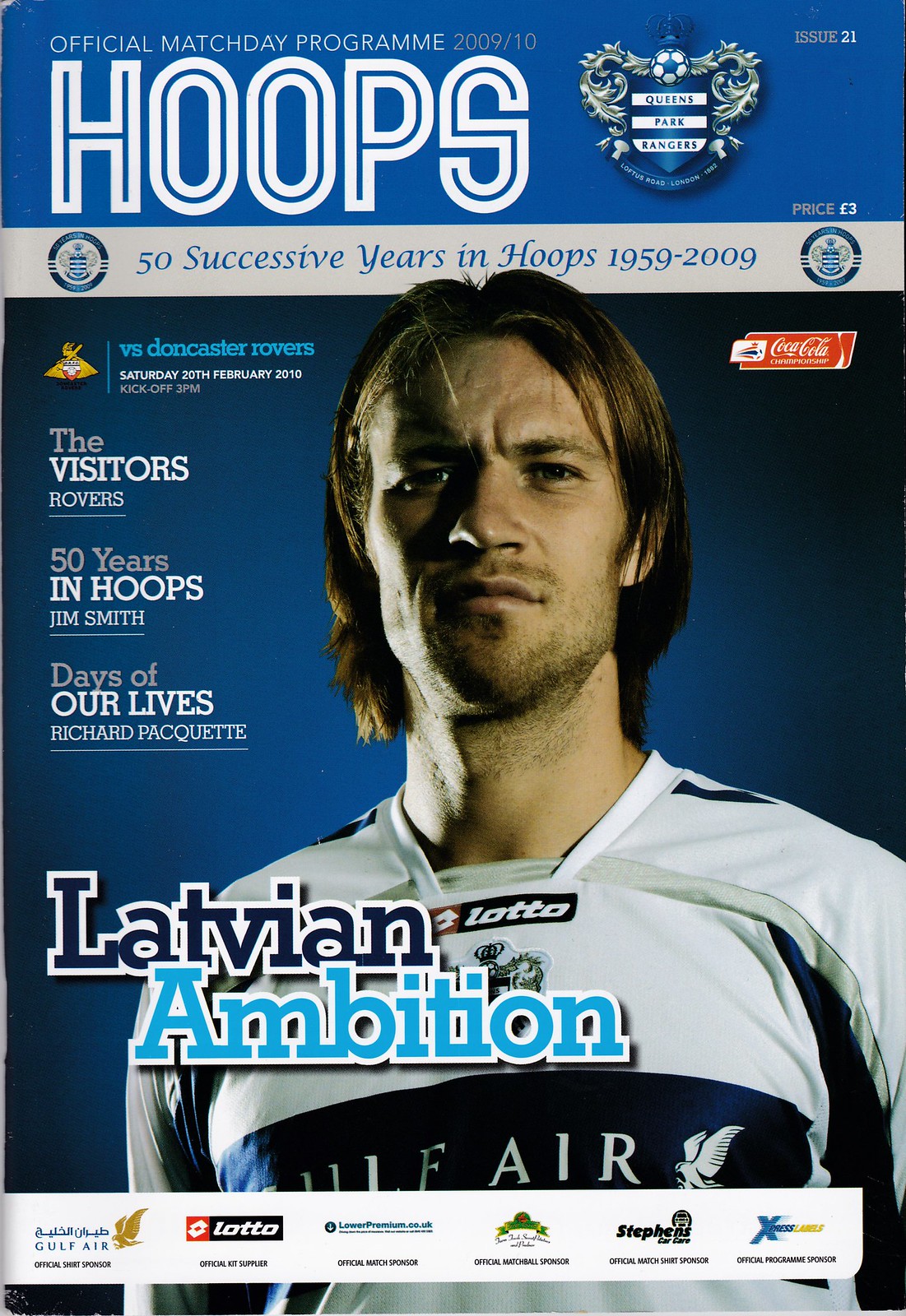The cover of the magazine features a bold blue background with white text that reads, "Official Match Day Program 2009-10." Centered prominently on the cover is a serious-looking football player with long, straight brown hair parted in the middle, wearing a white Gulf Air jersey with blue details and an eagle logo. The magazine highlights "Queens Park Rangers Issue 21" with the price listed as "European III." Below, a gray banner states "50 Successive Years in Hoops 1959-2009." Additional text includes "vs. Doncaster Rovers," with a kickoff date of "Saturday, 20th February, 2010, 3pm," and mentions of various features such as "Jim Smith," "Days of Our Lives," and "Richard Paquette." Over the player's image is a caption reading "Latvian Ambition." Several logos, including Coca-Cola, are featured towards the bottom alongside the text "The Visitors" and "Rovers, 50 Years in Hoops."